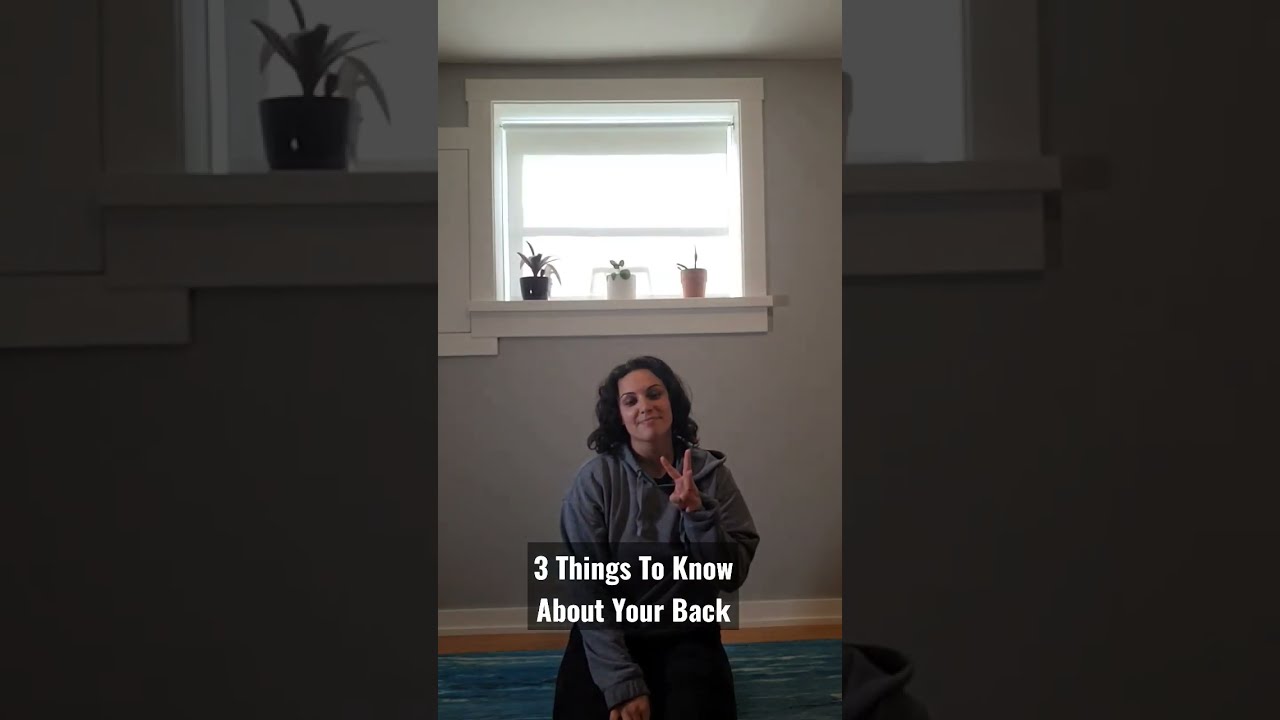The image is a meme featuring a young woman with dark hair kneeling on a blue carpet and smiling closed-mouthed at the viewer. She is wearing a blue hoodie and has one arm bent, showing what could be a peace sign or the number three. The central panel of the image includes two lines of white text against a black background, positioned near her left hand, reading, "Three things to know about your back." Behind her, a window with white trim lets in light, and a windowsill holds three potted plants in black, white, and terracotta planters. The meme uses a panel design where the left and right panels are close-ups of the windowsill and potted plants, creating cohesion and emphasis on the central theme. The wall behind her is gray with a white baseboard that meets a wooden floor, transitioning into the blue rug on which she is kneeling.